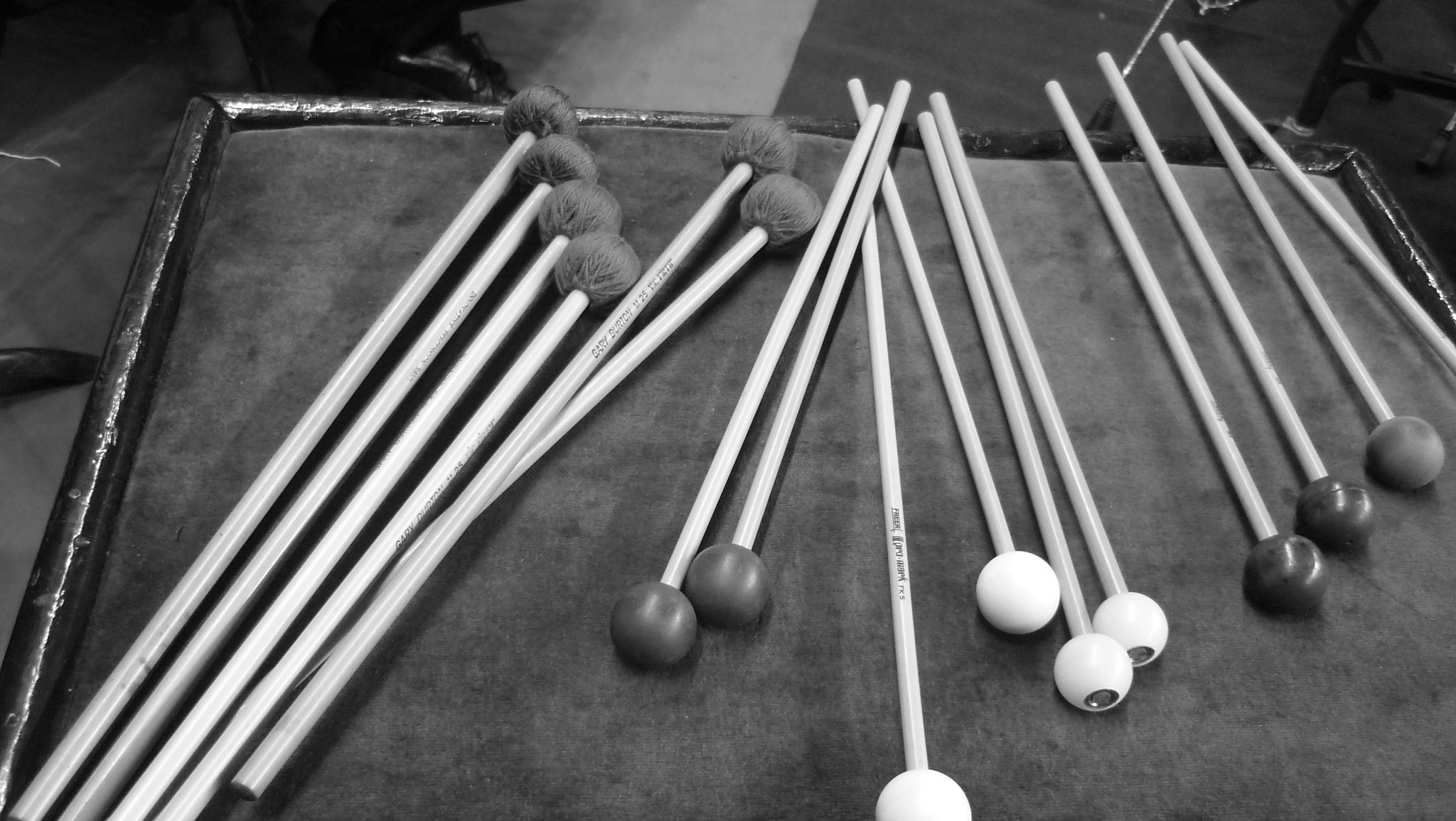This black-and-white photograph captures a scene in an orchestra pit, focusing on a large box with a wooden top, covered by a piece of velvet sound-deadening material. On this surface, various drumsticks—used for playing orchestral instruments such as large, round white drums—are meticulously arranged. These sticks are divided into three distinct groups: the first group, consisting of seven or eight sticks, has cloth pom-pom-like heads and features small black lettering on some handles. The second group, comprising six sticks, is notable for their reddish-colored rubber ball heads. Lastly, the third group includes four sticks with white, resin-like ball heads adorned with some form of writing. In the background, the scene includes a music stand and additional boxes, emphasizing the orchestral setting.